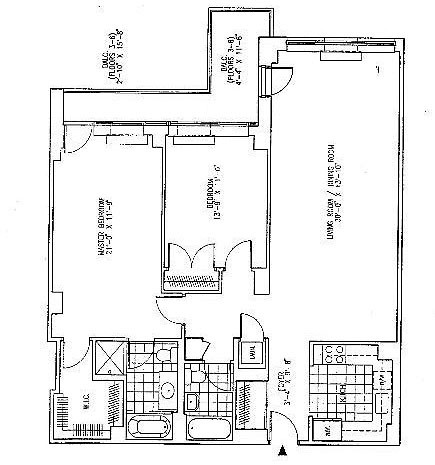Detailed Black-and-White Floor Plan of a Two-Bedroom Apartment:

This detailed blueprint-style floor plan of a two-bedroom apartment is presented in black and white with small, intricate writing. The layout reveals a thoughtfully organized living space with distinct areas. Upon entry, you are greeted by an interlay that leads directly to the living room. 

To the left of the entrance is a walk-in kitchen that is enclosed, offering a clear separation from the living room. Moving forward, the living room serves as the central hub of the apartment. Off to the left of the living room, there is a hallway that provides access to the first bathroom on the left and a bedroom on the right.

Continuing through the hallway, you will find the master bedroom. The master bedroom is equipped with a spacious walk-in closet and an adjoining master bathroom, offering additional privacy and convenience. 

Additionally, the living room opens up to a terrace on the left side, which extends in an L shape, providing outdoor space for relaxation. The overall aesthetic and detailed representation suggest that this is a photocopy of the original blueprint.